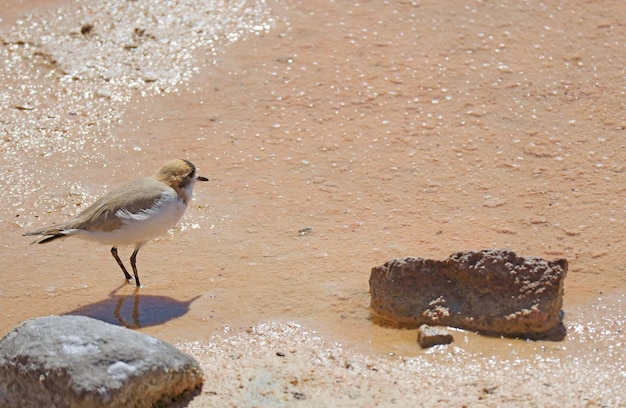The image depicts a bird on a beach, characterized by light-colored, gravelly, and sandy terrain with evident moisture, perhaps from recent rains or receding waves. Central to the scene is a large puddle, adding to the wet ambiance. The bird stands on the left side of the image, displaying a distinctive appearance with a white chest and belly, tan back feathers, a yellowy head, a black beak, and black legs. In the lower left corner of the image, there is a shoe-sized rock, and a similar rock appears towards the bottom right, enhancing the natural setting. The bird appears to be walking through shallow water, emphasizing the moist, tidal environment of the scene.